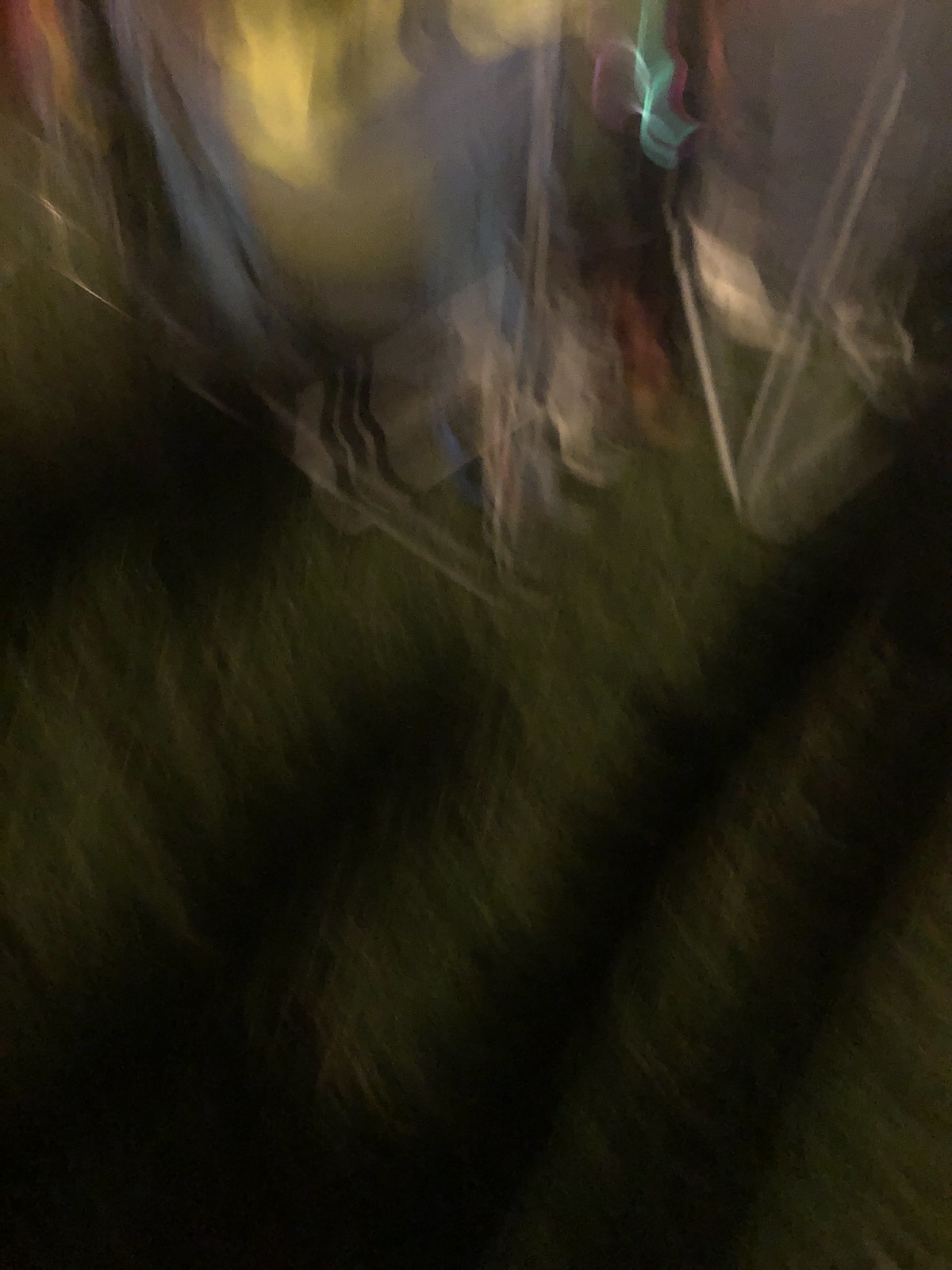A completely indistinct, blurred image features a chaotic mix of black, green, white, yellow, red, and aqua blue hues. In the upper left corner, a prominent yellow burst of light draws the eye, while an aqua burst similarly illuminates the upper right section. Scattered throughout, various sections of light and shadow create a dynamic interplay, contributing to the overall enigmatic atmosphere. White, V-shaped light patterns add a further element of intrigue. The lower half of the image is predominantly occupied by deep green and black tones, with hints of red subtly fading into the background.